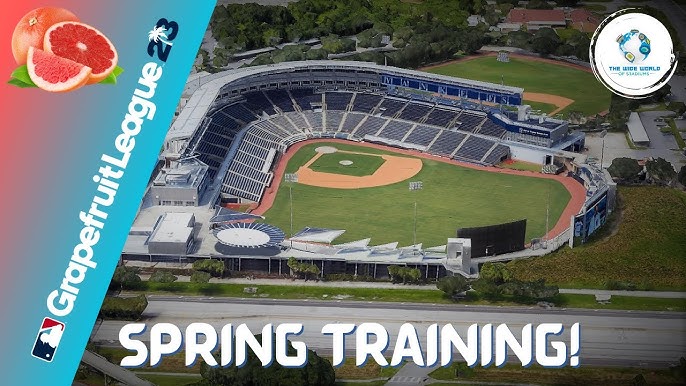The photograph, resembling an advertisement, features a baseball stadium at its center, surrounded by empty bleachers in a distinct upside-down U shape. The outfield and infield are vibrant green, while the diamond is composed of beige sand. Surrounding the ballpark are trees, and there's a road that runs in front of the stadium. In the upper left corner, a complex structure with a roof, the top of a building, and a large box air conditioner is visible, seemingly overlooking the field.

In the upper left corner of the image, there's an illustration of a whole grapefruit, a half grapefruit, and a slice, all adorned with green leafy sprigs. Adjacent to this is the text "Grapefruit League 23" in blue and red, flanked by the National Baseball Association (MLB) logo and a white palm tree situated between the numbers 2 and 3. 

At the bottom of the photograph, the words "Spring Training" are prominently displayed in white font. The image captures the sunlit field void of players, highlighting the serene yet anticipatory ambiance of the stadium ready for action.